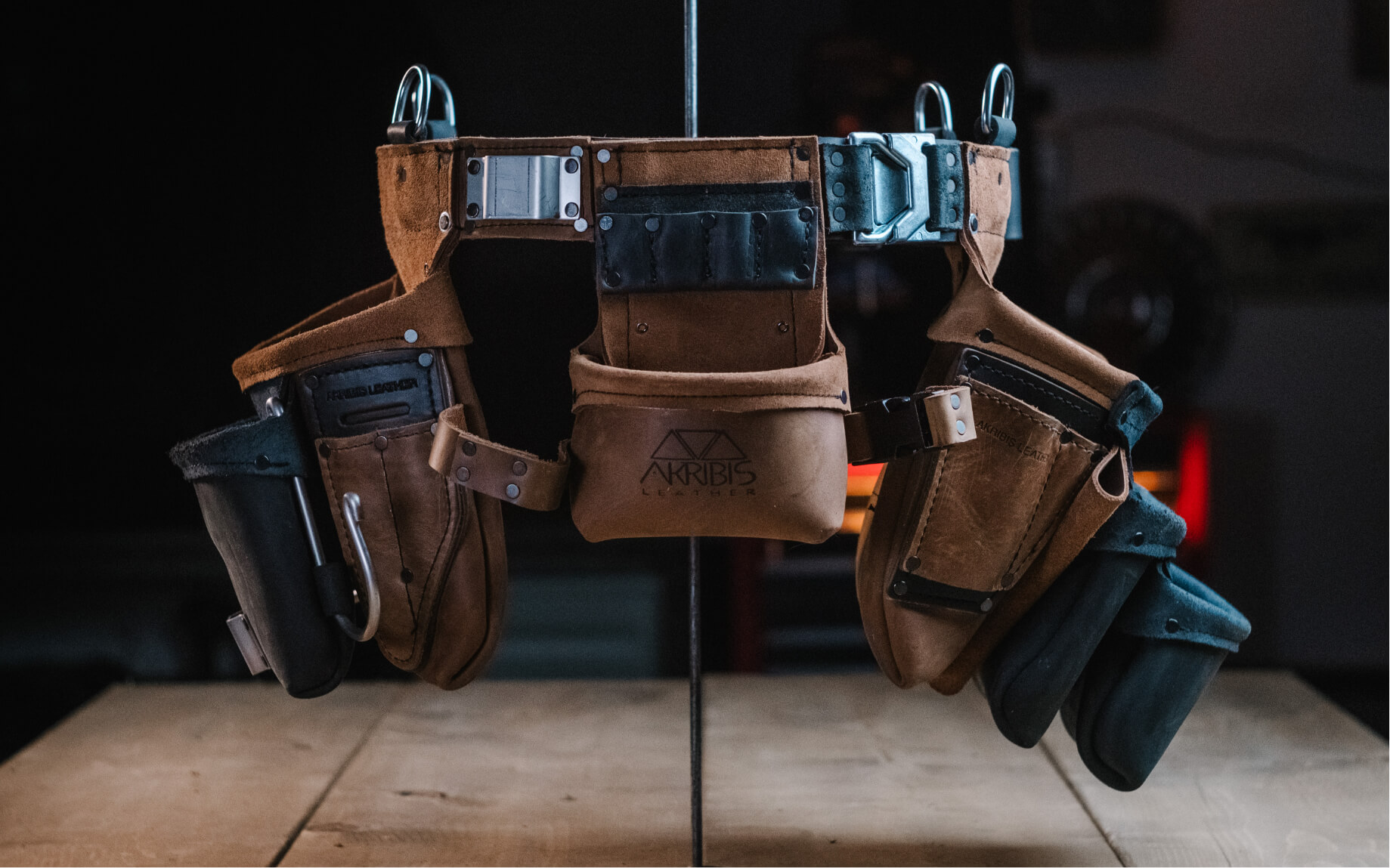The photograph depicts a meticulously crafted brown leather tool belt, prominently marked with the brand "Acribis Leather," featuring their distinctive triangle logos. This durable belt, designed primarily for utility, showcases an intricate array of pouches and compartments in both black and brown leather, ideal for storing various accessories or tools. Detailed rivets and robust stitching reinforce these pouches, while metal loops and hooks along the belt provide additional functionality for securing gear. The belt is suspended, giving a sense of it floating above a wooden surface, supported by a vertical metal rod extending from the table to the ceiling. The scene is set against a dark backdrop, emphasizing the tool belt's craftsmanship and versatility, making it suitable for work, hunting, or carrying an array of equipment.